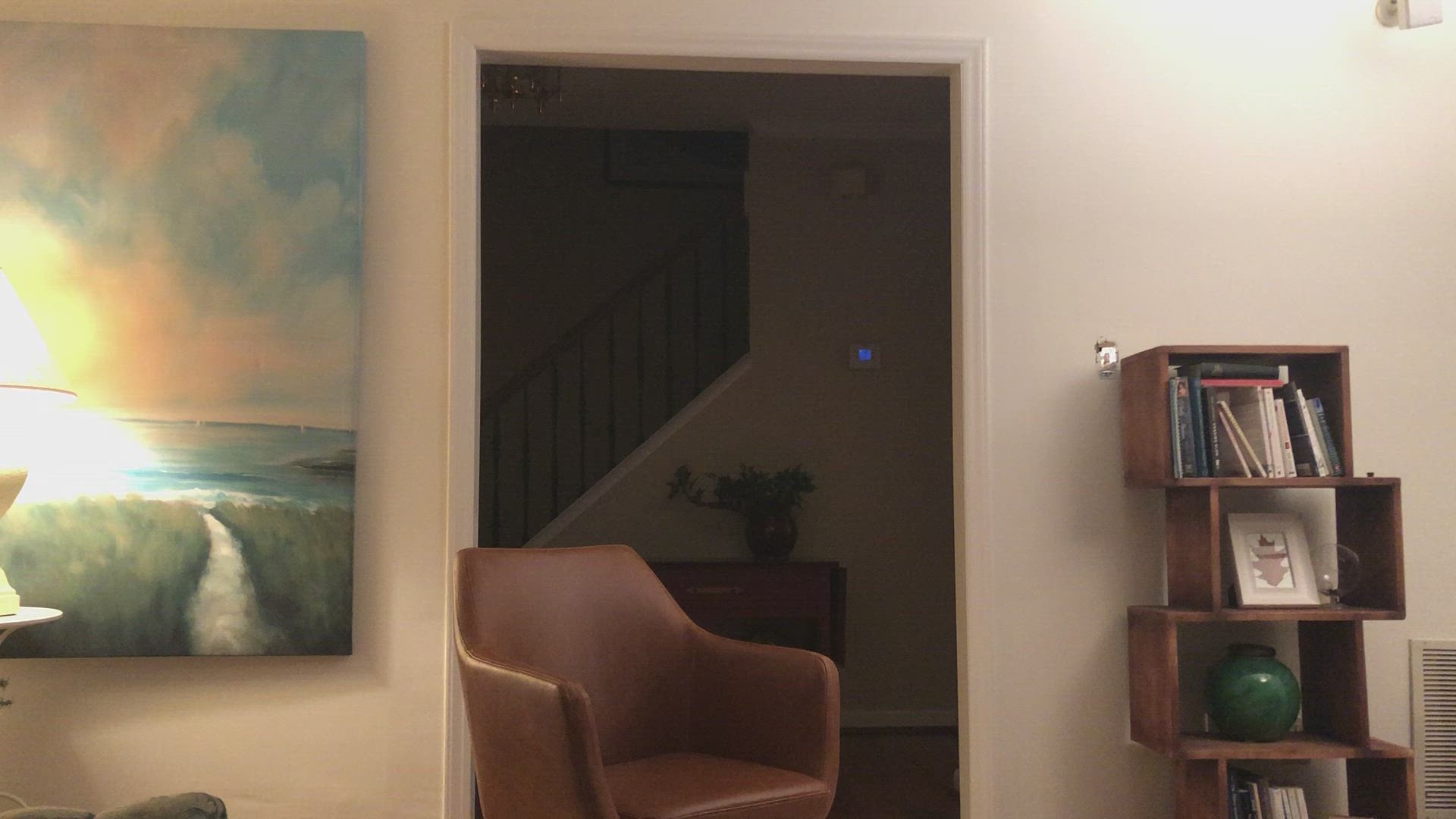In this realistic interior photograph of a house, the image captures two rooms divided by a door frame. In the background, through the door frame, a staircase ascends to the second story of the home, providing depth and a sense of dimension. In the foreground, the left side of the door frame features a painting hung on the wall, adding an artistic touch to the space. Sitting prominently in front of the door frame is a brown leather chair, suggesting a cozy seating area. To the right, against the wall, is a stacked, asymmetrical bookcase that holds an assortment of items, including books, a framed photo, and a distinctive green round glass vase, adding eclectic charm. The room is dimly lit, with a lamp on a small table illuminating part of the space, casting a warm glow on the painting and creating a cozy atmosphere.